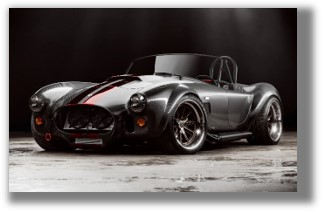The image showcases a sleek and modern-looking black two-door sports car, positioned prominently at the center of the frame. The car, possibly a small model or a full-sized vehicle, has an appearance that suggests it might be a Shelby Cobra, Porsche, or Jaguar. It's captured at a 45-degree angle from the front left, showcasing more of the driver's side than the passenger's side. 

The exterior features a striking crimson red and black racing stripe running down the middle of the hood, enhancing its sporty and racing appeal. The front of the car has a distinct bubbly design, particularly around the headlights, contributing to its classic yet modern look. The absence of the hood reveals a windshield and a unique circular metal piece at the back, adding to the detailed design. 

The car’s large, shiny wheels stand out against the almost marble-like or light gray concrete ground, which appears to be slightly moist. The entire scene is set against a black background with soft rays of light reflecting on the car’s surface, highlighting its polished finish and sleek curves. The photograph itself is horizontally oriented, emphasizing the expansive view of the car and its surroundings.